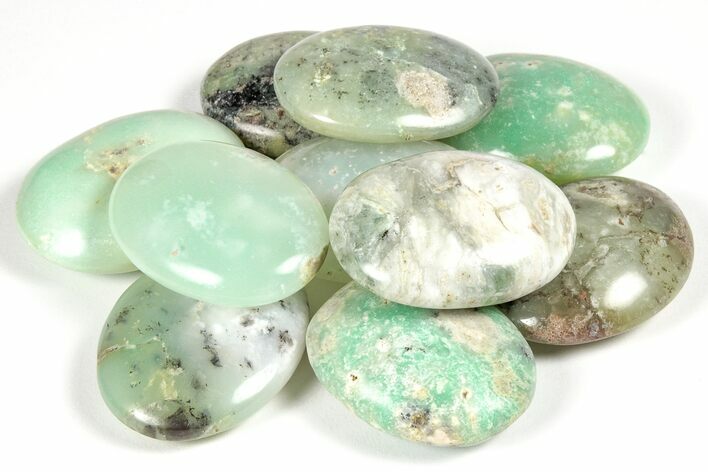This image is a close-up of a neatly arranged pile of round, smooth, and flat stones, resembling small flat eggs. The stones are stacked with a bottom layer of seven arranged in a circular pattern, and an additional three stones placed on top. Predominantly marbled in appearance, the stones exhibit a variety of colors; many showcase shades of light turquoise or aquamarine blue, while others display hues of gray, light green, and white, with some featuring dark patches or streaks of black. Each stone is highly polished, giving them a shiny and reflective surface. The arrangement is set against a clean, white background, highlighting their smooth textures and vibrant colors.